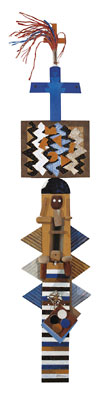The image is a detailed, totem pole-style piece of artwork with a distinctly claymation or cartoon-like texture. Starting at the bottom, the base is composed of bold stripes in beige, white, blue, and black. As one moves upward, about a third of the way up, triangular shapes appear, three on each side, each set of triangles aligned diagonally and colored differently on the left and right.

Above the triangles, a figure resembling a wooden doll stands, characterized by a brown face, black top, white eyes, curly wooden hair, and wooden legs. This figure has a black hat and is holding a tray with circular patterns in white, blue, brown, and rust colors along the rim.

Resting on the head of the doll is an abstract, rectangular artwork laid horizontally, featuring zigzag shapes in black, brown, white, orange, and blue. Above this rectangular artwork are two crosses: a larger blue cross at the base with blue and red streamers or ribbons flowing from it, partially covering the smaller orange cross with a tassel-like ornament on top.

The entire composition is topped by these two crosses, lending an intricate and multi-layered appearance to the image, blending elements of earthy wooden figures and vibrant abstract designs.